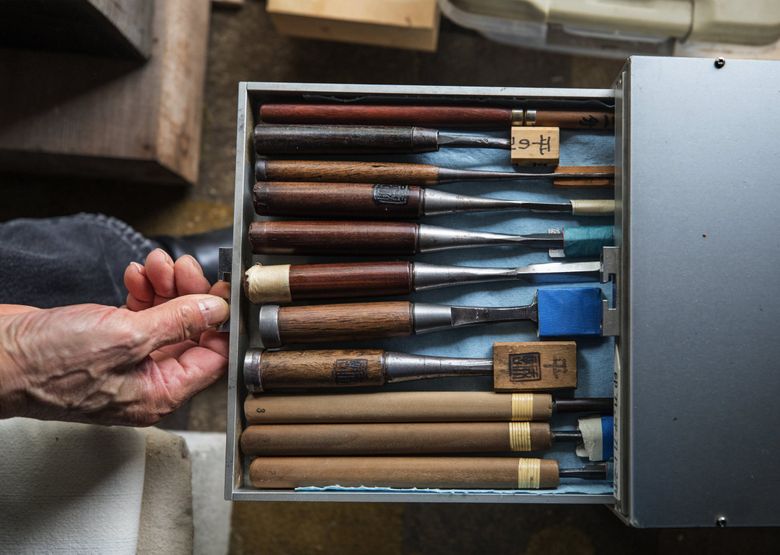In this image, we have a detailed view of a drawer being pulled open by an elderly individual. From a bird's eye perspective, you can see a wrinkled hand emerging from the left side, gripping the handle with their thumb and index finger, while their leg clad in black denim and a black leather shoe is partially visible. The drawer itself is a metal, silver-grey unit, possibly part of a filing cabinet, and is filled with 11 various tools, all neatly arranged. 

These tools, uniformly outfitted with wooden handles and varying in size, are organized across the entire drawer. Each tool has a distinctive appearance, some featuring a wooden block at the top and some exhibiting characters—possibly Japanese or Chinese—inscribed on them. These details suggest the tools might be related to printing. Despite the precise nature and possible cultural relevance of the characters, the exact function of each tool remains unclear. The drawer's interior features a blue covering underneath the tools, enhancing the overall orderly arrangement.